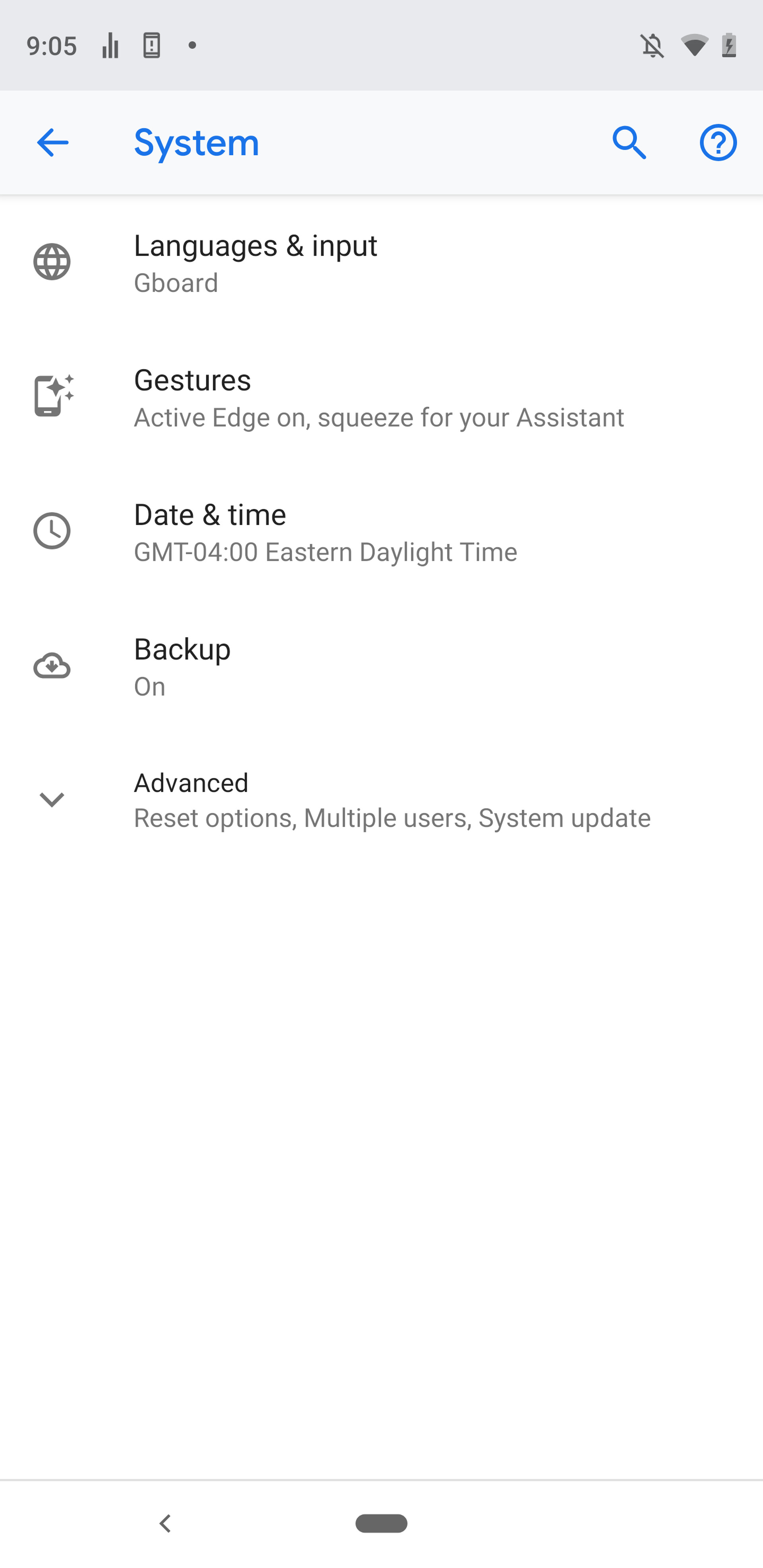The image displays a "System Settings" page on a mobile device with a white background. At the top, the word “System” is prominently featured in blue. Below this heading, a list of options is displayed in the following order: "Languages & Input," "Gestures," "Date & Time," "Backup," and "Advanced." 

In the upper left corner of the screen, the time is shown as 9:05, accompanied by a cellular signal icon. In the upper right corner, there are indicators displaying the phone's status, including a silent mode icon, a Wi-Fi signal, and a critically low battery level. The overall layout is straightforward and uncluttered, focusing solely on system configuration options.